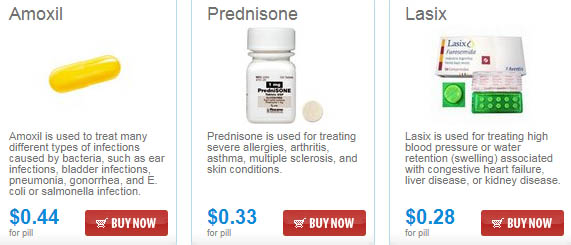In the image, three pharmaceutical products are prominently displayed. 

On the far left, there is a product named "Amozil." At the top of the Amozil product box, the name is clearly displayed alongside an image of a yellow pill positioned diagonally upwards. Below this, a detailed description reads: "Amozil is used to treat many different types of infections caused by bacteria, such as ear infections, bladder infections, pneumonia, gonorrhea, and E. coli or Salmonella infections." At the bottom left of this box, the price is indicated as 44 cents per pill, and a button marked "Buy Now" is located at the bottom right.

To the right of Amozil is a product called "Prednisone." The image associated with this product features a white bottle with a small circular pill shown to its right. The description states: "Prednisone is used for treating severe allergies, arthritis, asthma, multiple sclerosis, and skin conditions." The price is listed as 33 cents per pill.

The final product on display is "Lasix." The description for Lasix reads: "Lasix is used for treating high blood pressure or water retention associated with congestive heart failure, liver disease, or kidney disease." The cost is noted as 28 cents per pill. 

Each product is distinctively presented with its respective descriptions, uses, and pricing, offering potential buyers clear and concise information at a glance.